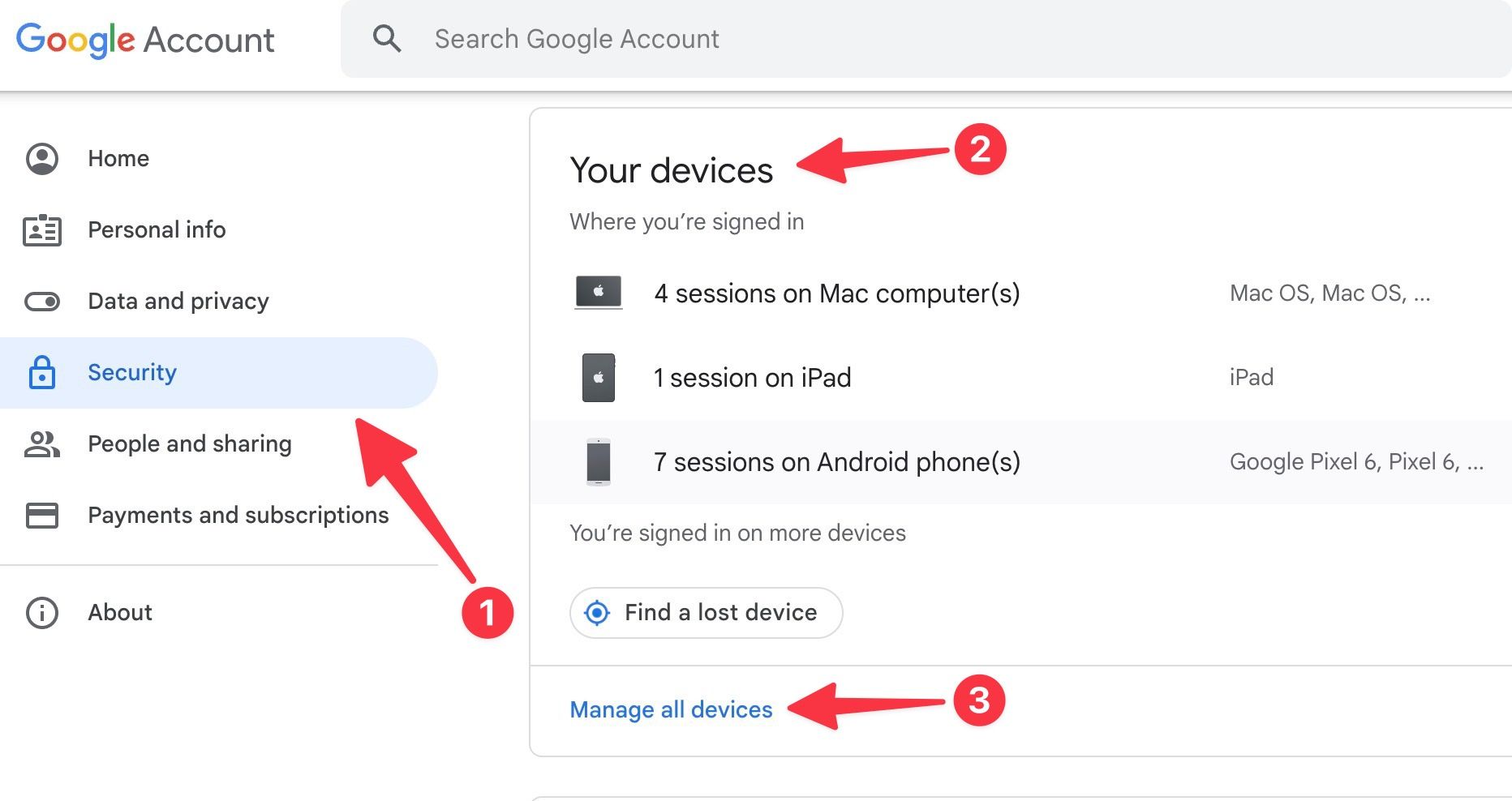The image predominantly features a white background with the Google logo in the upper left corner. The logo consists of the following colorful letters: "G" in blue, "o" in red, "o" in yellow, "g" in blue, "l" in green, and "e" in red, followed by the word "Account" in gray. Below the logo is a gray search box with a dark gray magnifying glass icon inside it, and the text "Search Google Account."

On the left-hand side, there is a vertical navigation menu with clickable tabs in black text. The tabs are labeled as follows:
- Home
- Personal info
- Data and privacy
- Security (highlighted in blue, indicating the current section being viewed)
- People and sharing
- Payments and subscriptions

A horizontal green-gray line runs across the interface, featuring an outlined circle with a lowercase "i" inside it in gray, and the word "About." A red arrow points to the "Security" tab, and at the other end of the arrow is a red circle containing the number "1" in white.

Further down the page, the content section is titled "Your devices" in black text, showing details about signed-in devices:
- 4 sessions on Mac computers
- 1 session on iPad
- 7 sessions on Android phones

The text "You're signed in on more devices" is displayed, followed by an oval button labeled "Find a lost device." At the bottom of this section, there is a blue button labeled "Manage all devices." A third red arrow points to this button, ending in a red circle with the number "3" in white.